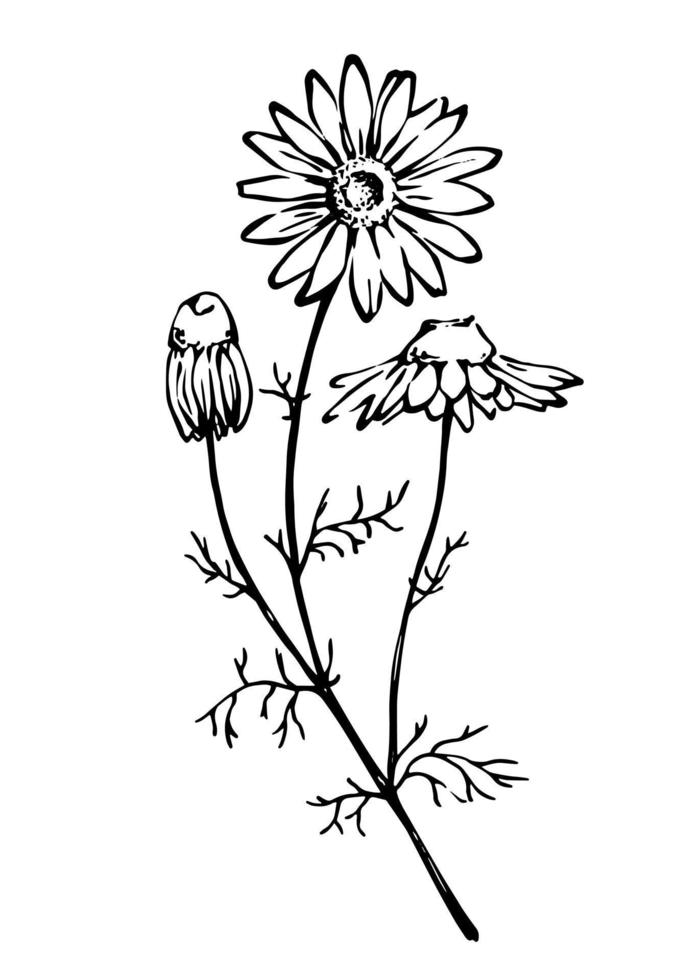This is a black and white drawing of a flower, rendered in a simple style. The image features a main stalk with two secondary stems branching off. The topmost stem holds a fully flowered bloom that appears to be a daisy, facing straight ahead. To the right, another bloom is slightly wilted and drooping downwards. On the left, a third bloom is completely wilted, with its petals hanging down and the bulb exposed. The entire composition lacks color and background, with the flower and its stems outlined against a plain white space. No fully formed leaves are present; only the outlines of leaf forms and some small branches are visible, giving the impression of a sparse and minimalist aesthetic. The sketch appears to be done with a black pen or marker, emphasizing the simple yet detailed representation of the flower and its different stages of bloom.